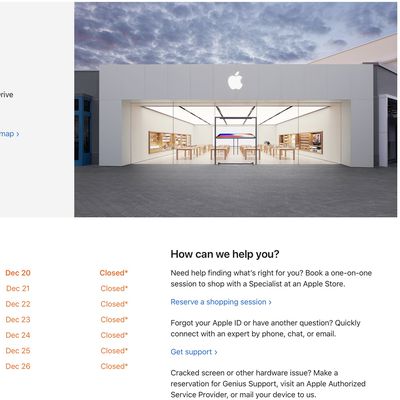This image is a detailed screenshot from a web page, likely from Apple, showing a small portion of the site. Central to the illustration is the depiction of an Apple Store. The store features a transparent facade, allowing a clear view of the interior where shelves line the walls and tables are arranged within the space. Dominating the upper part of the store's facade is the iconic white Apple logo. 

Beneath the store illustration is a text area set against a clean, white background. The first section reads, "How can we help you?" followed by an invitation to "Need help finding what's right for you? Book a one-on-one session to shop with a specialist at an Apple Store." This is complemented with a blue link that says "Reserve a shopping session" accompanied by a rightward-pointing arrow, indicating it is a clickable link.

Further down, there's an additional section addressing issues with an Apple ID or other questions: "Quickly connect with an expert by phone, chat, or email," followed by another blue link labeled "Get support." Additionally, a gray-font note mentions, "Cracked screen or other hardware issues? Make a reservation for Genius Support via an Apple Authorized Service Provider or mail your device to us."

To the left of this text, dates are listed in red: December 20th, marked as "Closed," and December 21st through December 26th, also indicating the store is closed on those dates.